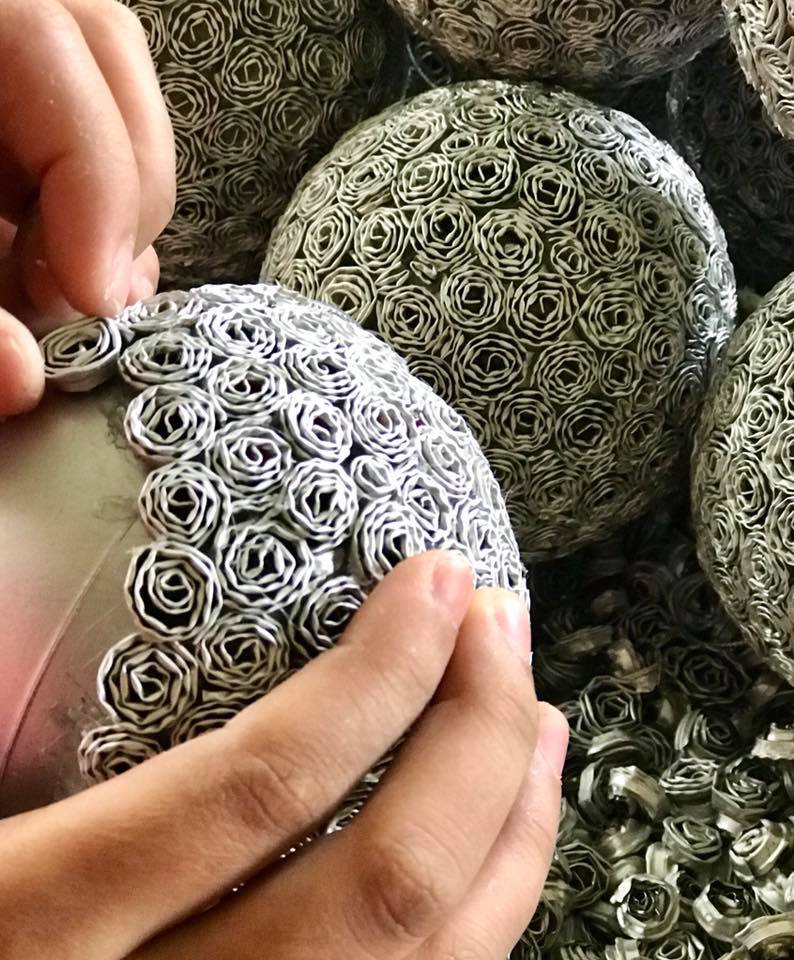In the image, a person is crafting ornate decorative spheres, meticulously adorned with small, snail-like fabric rosettes. Central to the scene are two delicate hands, their fingertips in action, affixing a rosette onto a large white ball. The fabric rosettes, in a gradient of silvery hues—ranging from white to gray to black—cover the sphere in intricate, coiled patterns, reminiscent of roses. Below the hands lies a collection of these intricate rosettes, presumably awaiting attachment. The repetitive, detailed handiwork suggests a time-consuming process, emphasizing the dedication and precision needed to embellish each sphere.